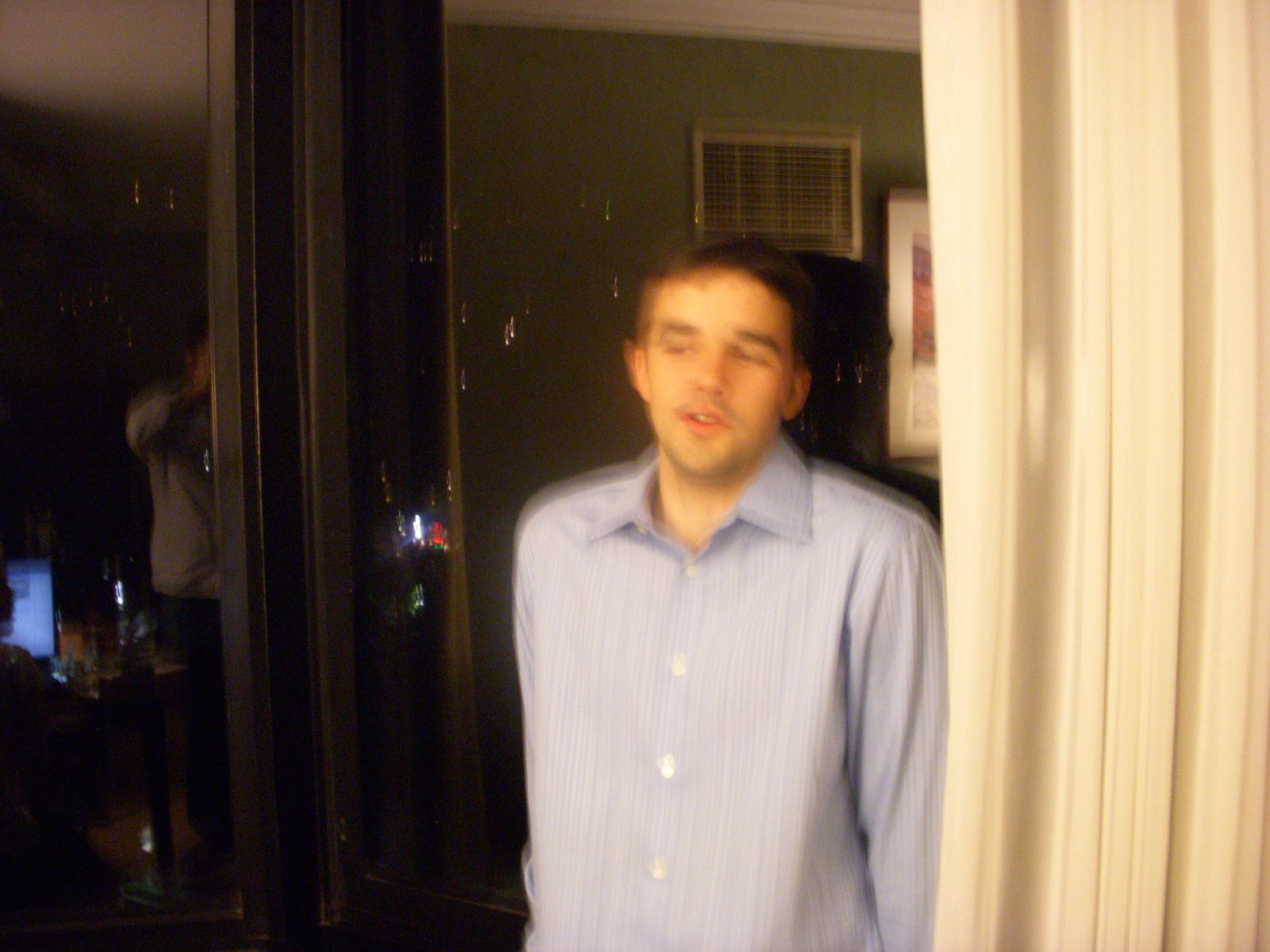This is a color snapshot of a young man in his 20s, centrally positioned within a square frame. He’s wearing a long-sleeve light blue shirt with buttons and gazes off to the right. To his left, a mirror reflects both the person taking the photograph and another individual seated at a computer. The computer sits open on a table. Behind the man, the background features a dark green wall with some paint drips, adding a textured look that might be mistaken for stains on the photo. There's also a small picture mounted on the wall, catching some light reflections. The right-hand quarter of the frame shows either a white curtain or white plastic doors. Additionally, behind the reflection, faint lights resembling those from businesses are visible, adding depth to the composition.